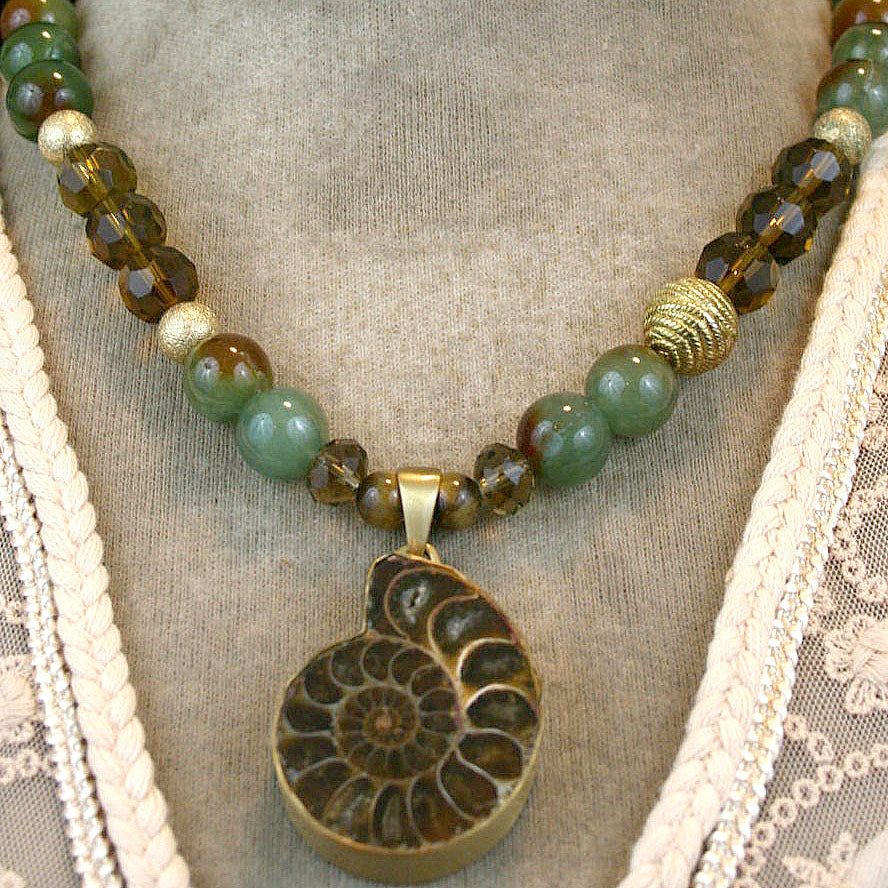The image displays a close-up of an intricate, artsy necklace draped on a gray mannequin, adorned with a white lacy blouse featuring a V-neck with braided edging. The necklace itself is composed of various kinds and sizes of beads, including large emerald green beads speckled with brown, smaller semi-translucent amber beads, and roughened gold beads, interspersed in a repeated pattern. At the center hangs an authentic-looking ammonite shell pendant, attached with a gold hook and clasp. The pendant, resembling a cut lengthwise snail's shell with ridges, adds a unique, swirly medallion look that is both elegant and symbolic.